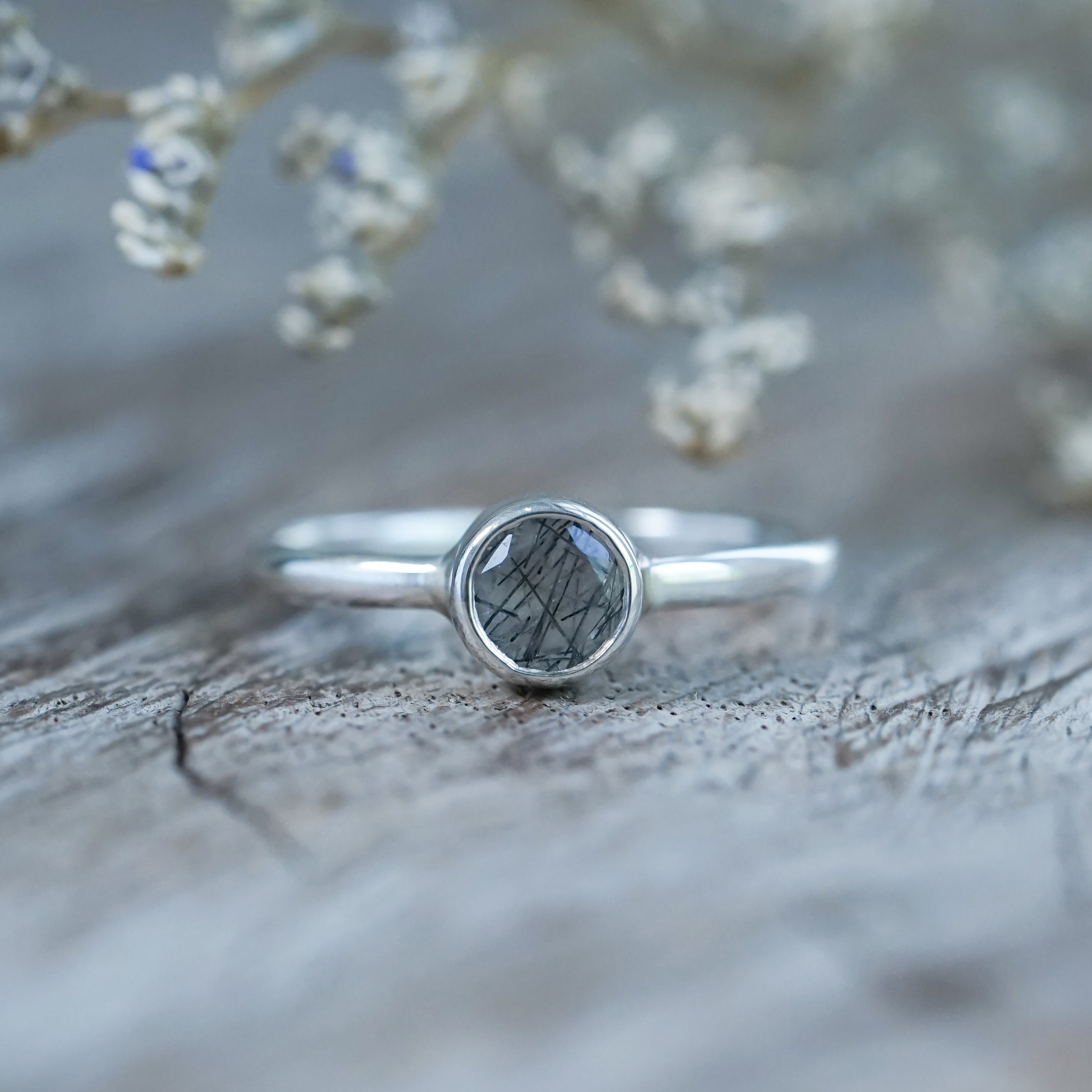This close-up photograph features a silver ring prominently placed on a slightly blurred surface. At the center of the ring is a round, light green stone interspersed with random black squiggly lines, giving it a unique, glass-like appearance. The bottom and top edges of the image are blurred, with the upper part featuring another piece of blurred jewelry that exhibits both silver and blue elements. The surface on which the ring rests appears to be metallic gray or silver, and there is a small, indistinct black object near the ring. The entire photograph is almost square in shape, capturing a detailed and elegant view of what appears to be a lady's ring amidst other metallic and jewel-toned accessories.